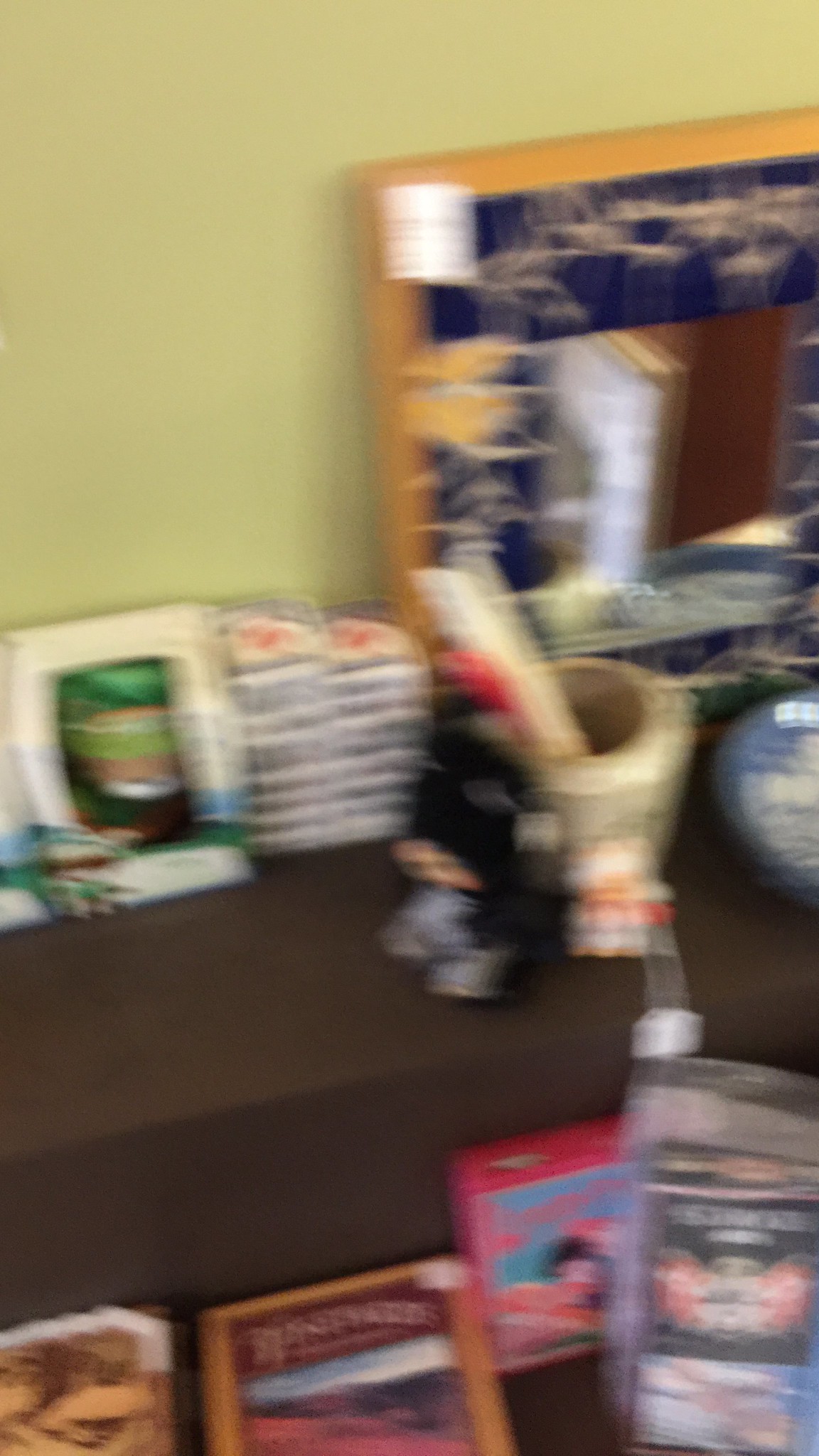A blurry, out-of-focus indoor photo depicting a cluttered desk laden with various items and knickknacks. The background features a pale yellow wall, giving the scene a warm ambiance. The desk is cluttered with an eclectic mix of objects, hinting that this could be a store. Whiter spots among the items could be sale tags, suggesting the items are for sale. Prominently placed in the background is a square mirror with a stained glass rim, leaning against the wall. A mortar and pestle can be observed amidst the chaos. On the floor, ornate boxes and signs are scattered. Some unidentifiable objects are strewn across the desk and concentrated on the right side. The overall scene is a hodgepodge of curiosities and decorative pieces, adding to its intriguing but chaotic nature.